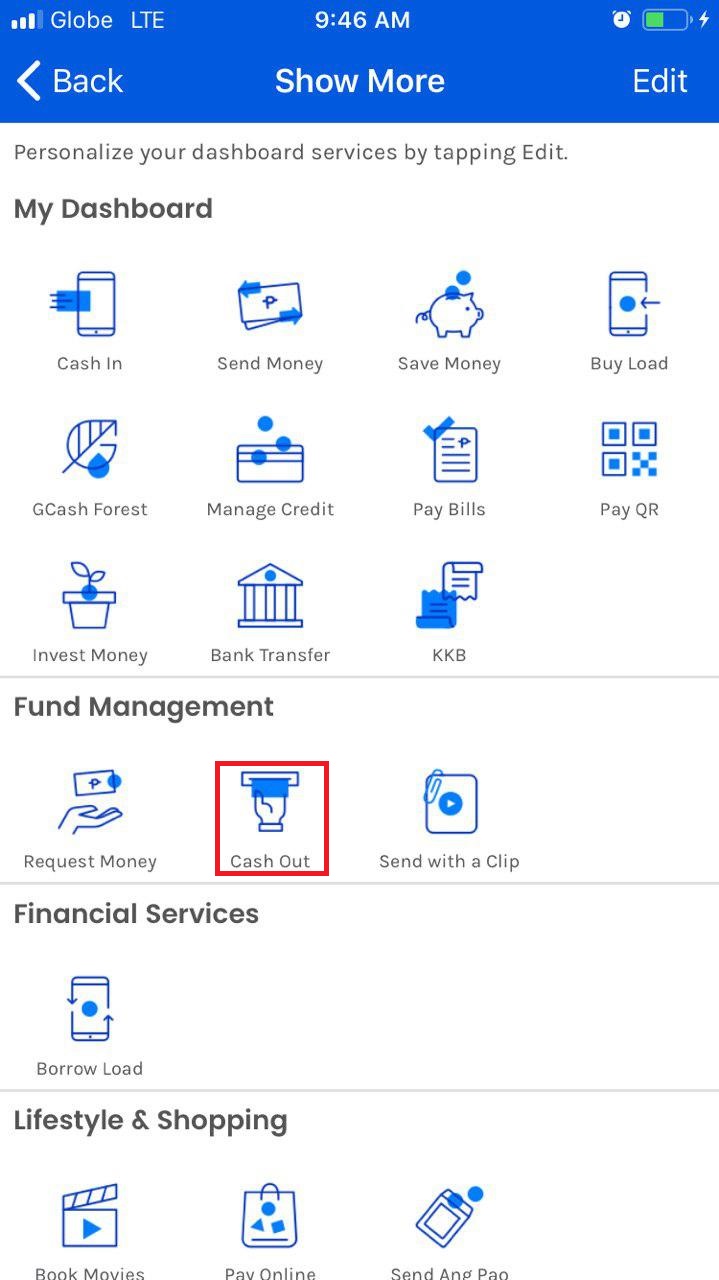Here is a detailed and cleaned-up descriptive caption based on the provided content:

---

The screenshot captures a webpage with a distinctive blue header prominently displaying the title "Show More" in the center. On the left side of the header, there is a back button or icon, while an "Edit" text is positioned on the right. The webpage itself has a clean, white background and is organized into five distinct sections, each divided by a line.

Directly below the blue header, there is a small instructional text that reads, "Personalize your dashboard services by tapping Edit." The first section beneath this text is labeled "My Dashboard," featuring around twelve icons. These include:
- "Cash In" icon
- "Send Money" icon
- "Save Money" icon
- "Invest Money" icon, depicted by a potted plant
- "Bank Transfer" icon, illustrated by a bank facade
- "KKB" icon, represented by two documents

Following the "My Dashboard" section is the "Fund Management" section, which contains three icons:
- "Request Money"
- "Cash Out," depicted by an icon of a hand retrieving money from a dispenser, boxed in red
- "Send with a Clip"

The third section is "Financial Services," which includes a single icon labeled "Borrow Load."

The final section, "Lifestyle and Shopping," comprises three icons:
- A "Book Movies" icon
- A "Pay Online" icon
- A "Send ANGPAO" icon

Each section and icon is distinctly organized, enabling easy navigation and personalization of the dashboard based on user preferences.